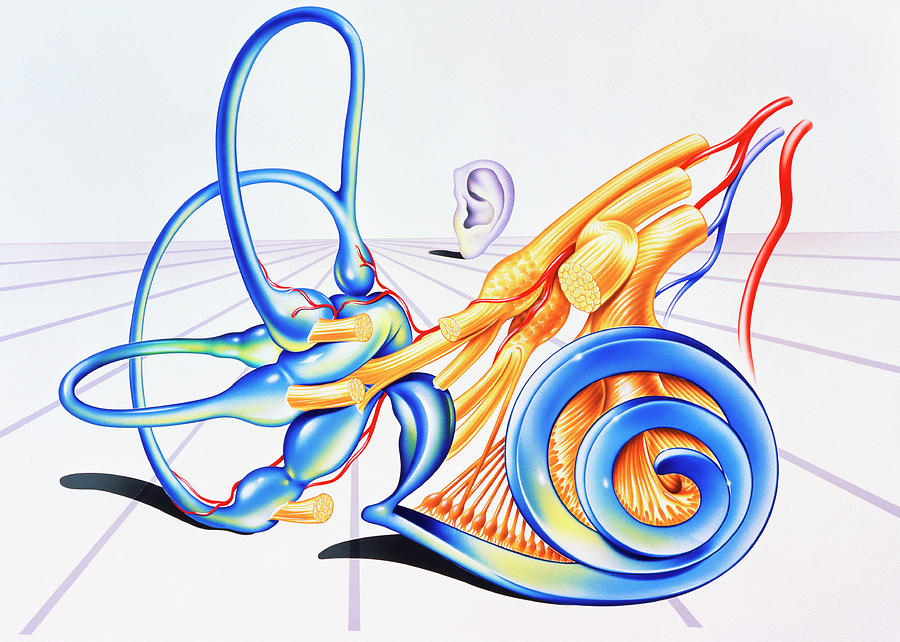The image is a detailed and vivid digital artwork, visually striking and rich in color. In the background, centrally-positioned and subtly illustrated, is a drawing of an ear, specifically the earlobe, devoid of any facial context. Foregrounding the piece is a compelling and intricate graphic of what appears to be the inner ear, prominently featuring parts such as the cochlea, nerves, and semicircular ducts. This inner ear section is rendered in vibrant hues of blue, yellow, red, and accented with some green, effectively drawing the viewer’s attention. The off-white plane on which the structures are set is interspersed with light purple lines that guide the eye towards the back, adding depth to the image. While the precise anatomical elements are challenging to identify without labels, the artwork superbly blends conceptual flair with a semblance of scientific diagramming, focusing heavily on the inner workings of the ear.